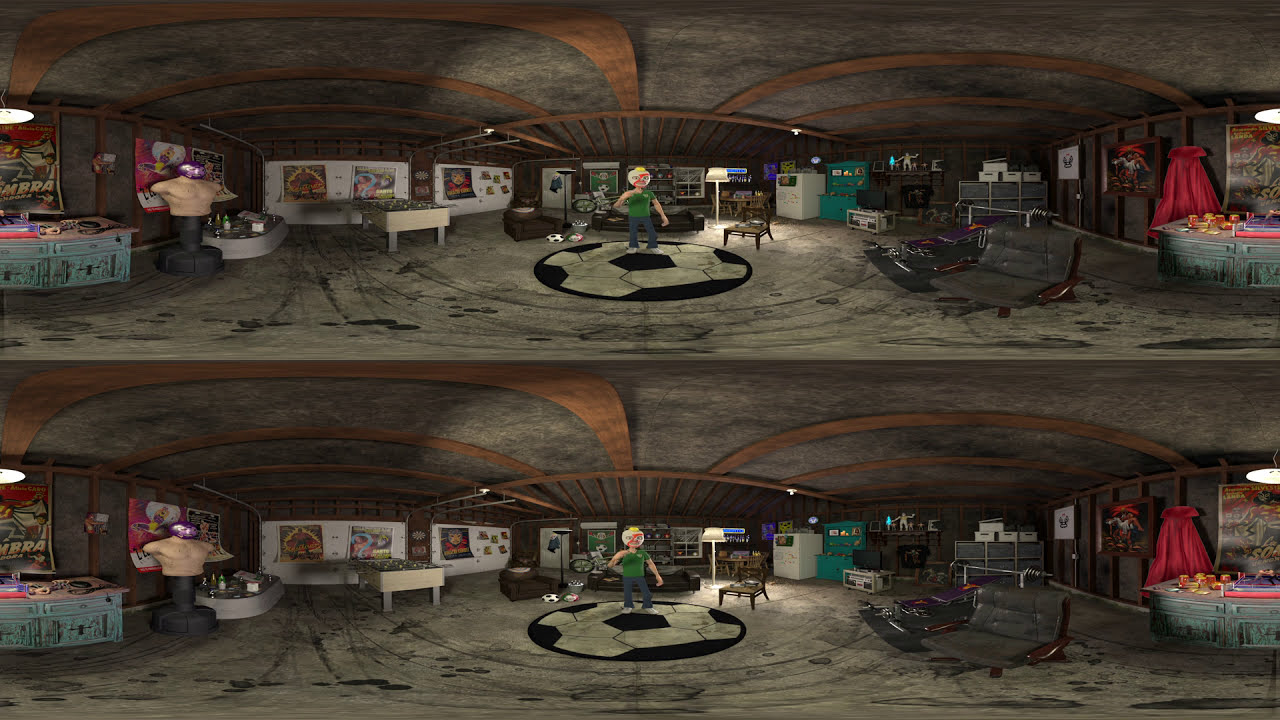The image depicts a computer-generated scene, likely from a virtual reality video game. It features a wide, panoramic, 360-degree view, displayed in a split-screen format with the same image mirrored on the top and bottom halves. The setting resembles a man cave or a game room, possibly located in a basement or a garage, given the dingy concrete floor marked with oil stains and streaks, and a ceiling made up of concrete and wooden beams.

Central to the scene is a male character wearing a green shirt, blue jeans, and a luchador wrestling mask, standing on a circular rug designed to look like a soccer ball. The room is furnished with various items that contribute to the man cave ambiance: a foosball table, a white piano or table, a living room lamp, several chairs and couches, and posters on the walls that depict soccer games and Mexican wrestlers. Additionally, there appears to be a wrestling dummy on the left-hand side, contributing to the rugged theme of the space. The character seems to be posing for the camera, enhancing the lifelike, immersive qualities of this animated, virtual environment.